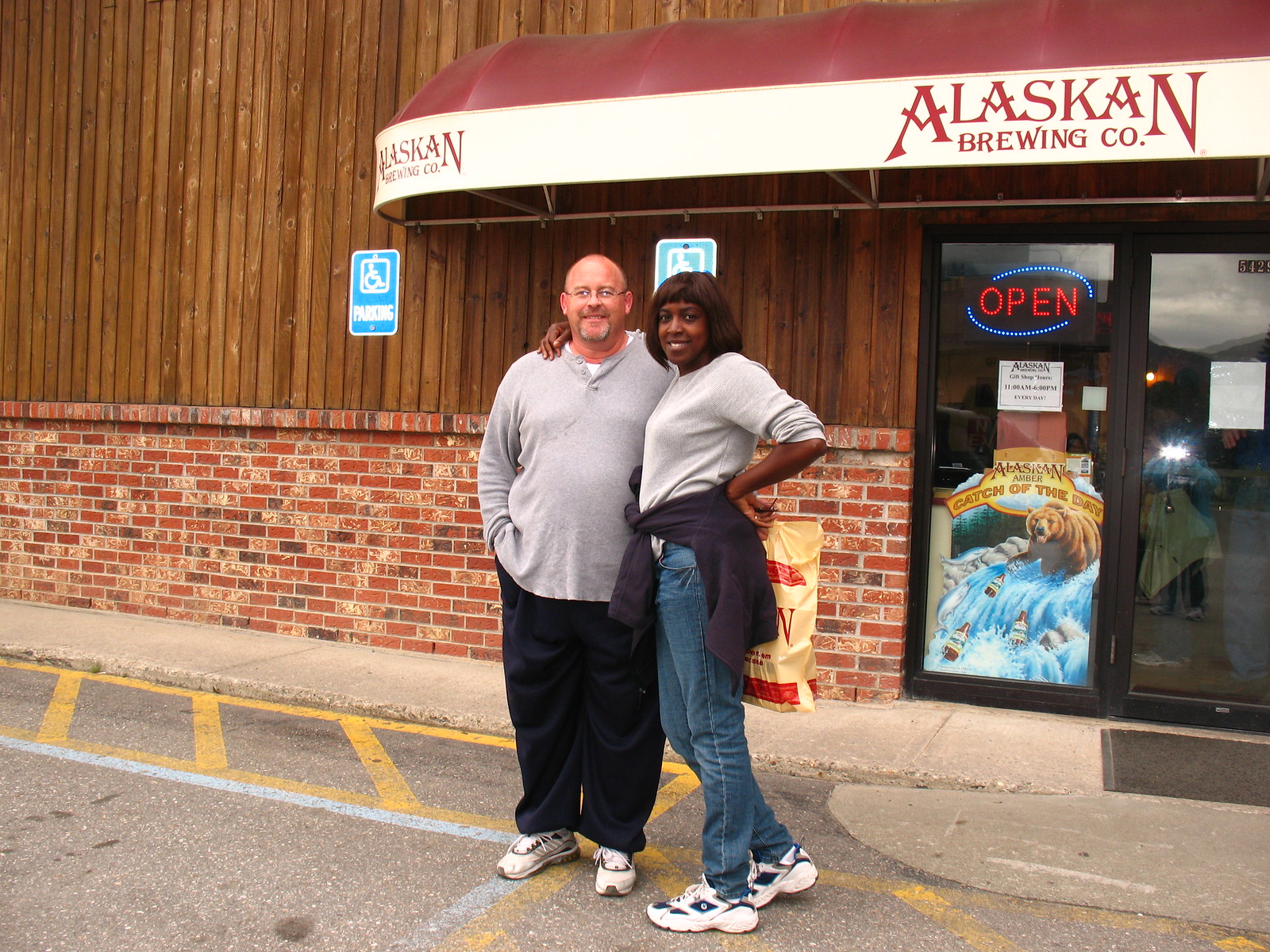In this rectangular photograph, we observe a moment captured outside the Alaskan Brewing Company. The backdrop features a distinctive building with a four-foot-high brick base in hues of red, brown, and black, topped with medium to dark-stained vertical wood paneling. An illuminated "Open" sign and glass doors reflect the flash of the photographer's camera, adding a lively touch. The architectural elements also include a prominent red and white awning bearing the company name. Yellow and white lines on the ground hint at the parking lot setting, complete with two handicap parking signs affixed to the wall.

At the center of the image stand a black woman and a white man, both smiling and posing for the camera. The woman has shoulder-length brown hair and is dressed in a gray long-sleeve shirt, blue jeans, and sneakers. A purple hoodie is tied around her waist, and she holds a brown plastic sack in her hand, with one arm around the man and her other hand on her hip. The man, a bit on the heavier side and wearing glasses, sports a gray long-sleeve shirt over a white undershirt, dark pants, and tennis shoes. Together, they exude a sense of camaraderie and joy, commemorating their visit to the Alaskan Brewing Company.